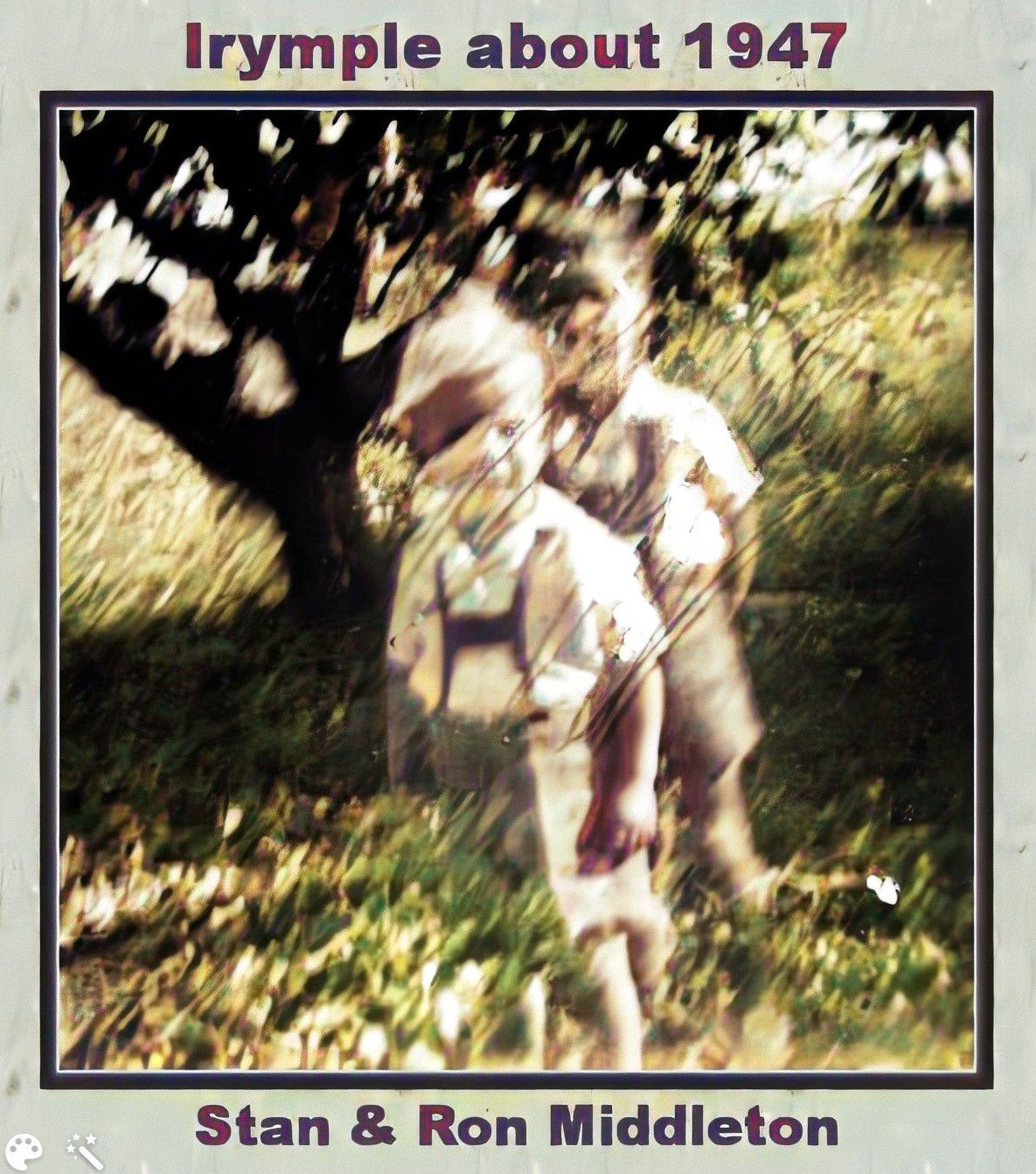This vintage photograph, encased in a green border with a darker black inner frame, captures a nostalgic moment from around 1947. The image shows two young boys, identified as Stan and Ron Middleton, standing in a verdant field beneath the shade of a leafy tree with a brown trunk. Both boys, possibly around six or seven years old, are dressed in white short-sleeved button-up shirts, green shorts, and dark brown suspenders, reminiscent of traditional lederhosen attire. Though the photo is slightly blurry and the figures appear almost ghostly, giving the impression of a bygone era, the handwritten text adds a poignant touch: "Irymple, about 1947" at the top and "Stan and Ron Middleton" at the bottom.